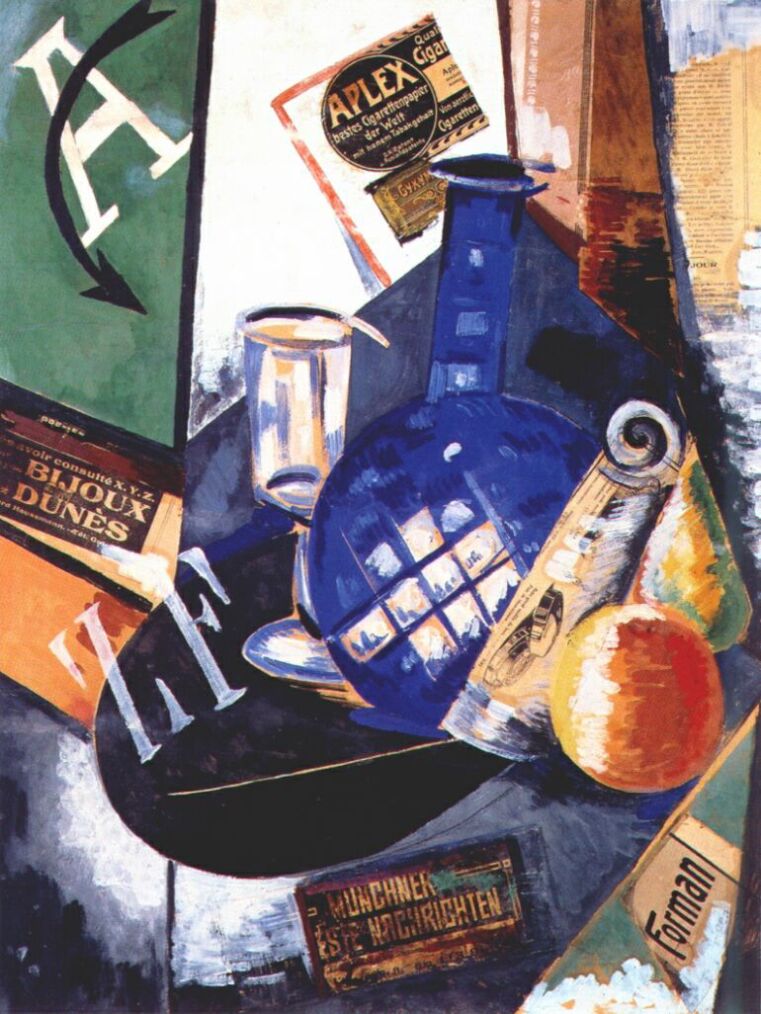In this modern and visually busy painting, a diverse collage of objects and colors is depicted against a dynamic background that transitions from black, blue, and gray hues. Centrally, an array of eclectic items appears to be arranged on a table: prominently featured is a tall, blue vessel resembling either a bong or a glass with a long neck, flanked by fruit, possibly an orange, and a variety of geometrical still-life objects in oranges, greens, and yellows.

Scattered across the scene are fragments of torn labels and faded newspaper clippings, adding to the chaotic collage effect. These labels contain words and phrases in various languages, such as "Bijoux Dunes," "Aplex," "Foreman," "Munchen Este," and "ZF." Notably, a curved arrow overlays the letter "A," contributing to the modern and daring aesthetic of the piece.

Amid the clutter of packages, containers, and abstract forms, a pennant with daisies and an object that might be a test tube or horn lend further ambiguity to the composition. In the upper right, a torn news clipping dangles as if affixed to a wall. The intricate array of objects might suggest a setting, perhaps a table in a window of a coffee shop, with background elements like clouds and a distant tree line subtly integrated into the periphery.